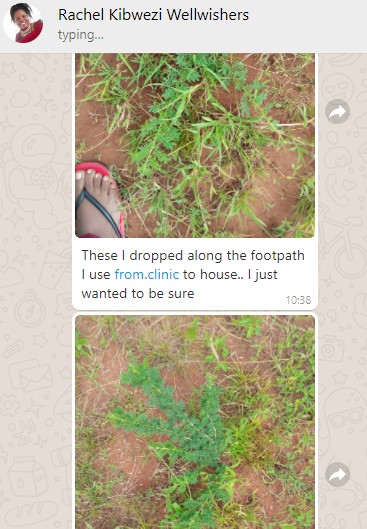The image is a screenshot from a WhatsApp conversation with Rachel Kibwizi Wellwishers. At the top left corner of the screen, there's a profile picture of Rachel, a black woman wearing a red dress. Her name is displayed next to the picture, and her status indicates she is typing. The chat window shows a timestamp of 10:38. 

The conversation includes two images taken from ground level. The first image shows Rachel's right foot in a flip-flop with black straps and a red bottom, placed on the left side of the image. The ground beneath her foot is muddy with some greenery, possibly weeds or plants. The second image mostly shows the muddy ground with more greenery, likely taken along the footpath she mentions. Rachel has written a message saying, "These I dropped along the footpath I used from clinic to house. I just wanted to be sure." The WhatsApp app interface includes icons of a phone and a bicycle against a grey background with little stars, adding to the familiar feel of the messaging platform.